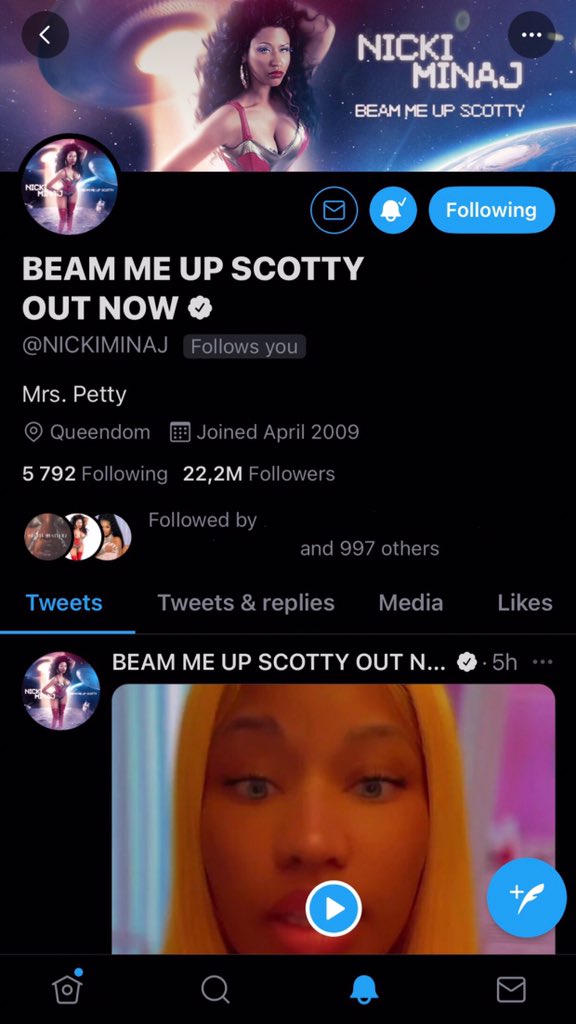This image showcases a screenshot of Nicki Minaj's verified Twitter profile, captured from a mobile device. At the top of the page, there's a back arrow on the left and a list button on the right. The header features cover art for her release, "Beam Me Up, Scotty," prominently displaying the text "Nicki Minaj, Beam Me Up, Scotty, Out Now" against a sleek black background.

Nicki Minaj's profile includes a verified blue check mark beside her handle, @NickiMinaj, and an indication that she follows the account viewing this profile ("Follows You"). Further details reveal that she joined Twitter in April 2009. She is following 5,792 accounts and boasts 22.2 million followers.

Below these details, there are navigation tabs for viewing her tweets, tweets and replies, media, and likes. A video player is visible at the very bottom of the screen, suggesting there is a video available for viewing on her profile.